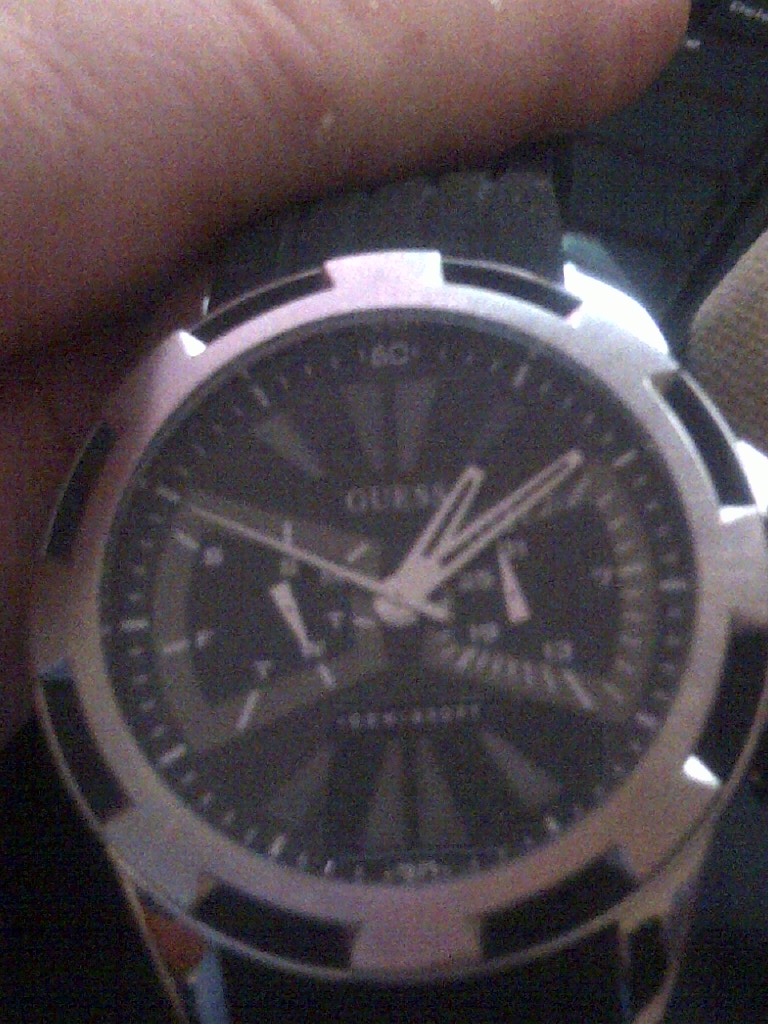This close-up photograph showcases an older-style, round GUESS wristwatch. The watch features a silver case with rectangular indentations along its outer edge, providing added detail. The black watch face prominently displays the brand name "GUESS" and includes some highlighted sections and gray markings. The time on the watch reads 1:09 and 4.50 seconds, indicated by its white hands. The watch band appears to be made of black cloth. At the very top of the image, a part of a person's finger is visible, suggesting they are holding the watch.